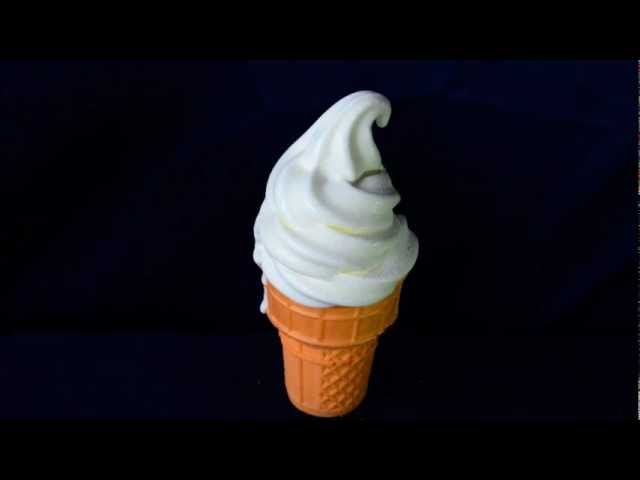This photograph features a cylindrical ice cream cone with a flat bottom and intricate latticework and grid patterns on its light brown, wafer-like surface. The cone is topped with a thick swirl of creamy white vanilla ice cream, crowned by a neatly curled peak that tips slightly to the right. White drips on the left side of the ice cream indicate slight melting, adding a touch of realism to the scene. Set against a solid black background that highlights its features and gives the impression of floating in a void, the ice cream cone is illuminated, adding a slight reflective sheen to the vanilla ice cream. The simplicity of the black backdrop accentuates the central positioning and detail of the cone, making it the focal point of the image.